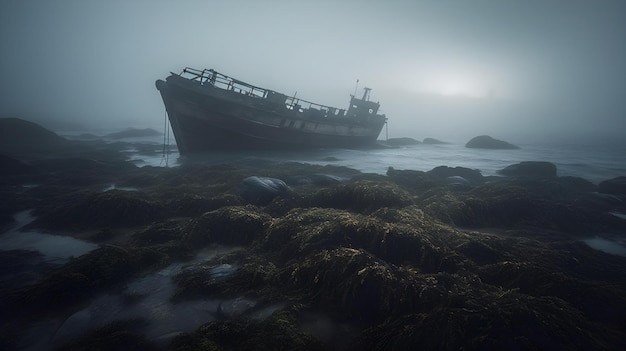This image captures a misty coastal scene during what appears to be an early morning shrouded in fog. The dim light, possibly from a faint, rising sun barely visible through the upper right-hand corner of the fog, gives the environment a hazy and ethereal ambiance. The shoreline is scattered with numerous brown, seaweed-covered rocks, enhancing the rugged essence of the location. Dominating the mid-ground is a large, dark-colored, industrial ship with a distinctive double white stripe on its side. The vessel, appearing weathered and rusted, rests at an awkward angle as it has clearly run aground on the rocky shore. The ship’s deserted and time-worn state suggests it has been stranded here for quite some time, adding a poignant touch to the maritime landscape.